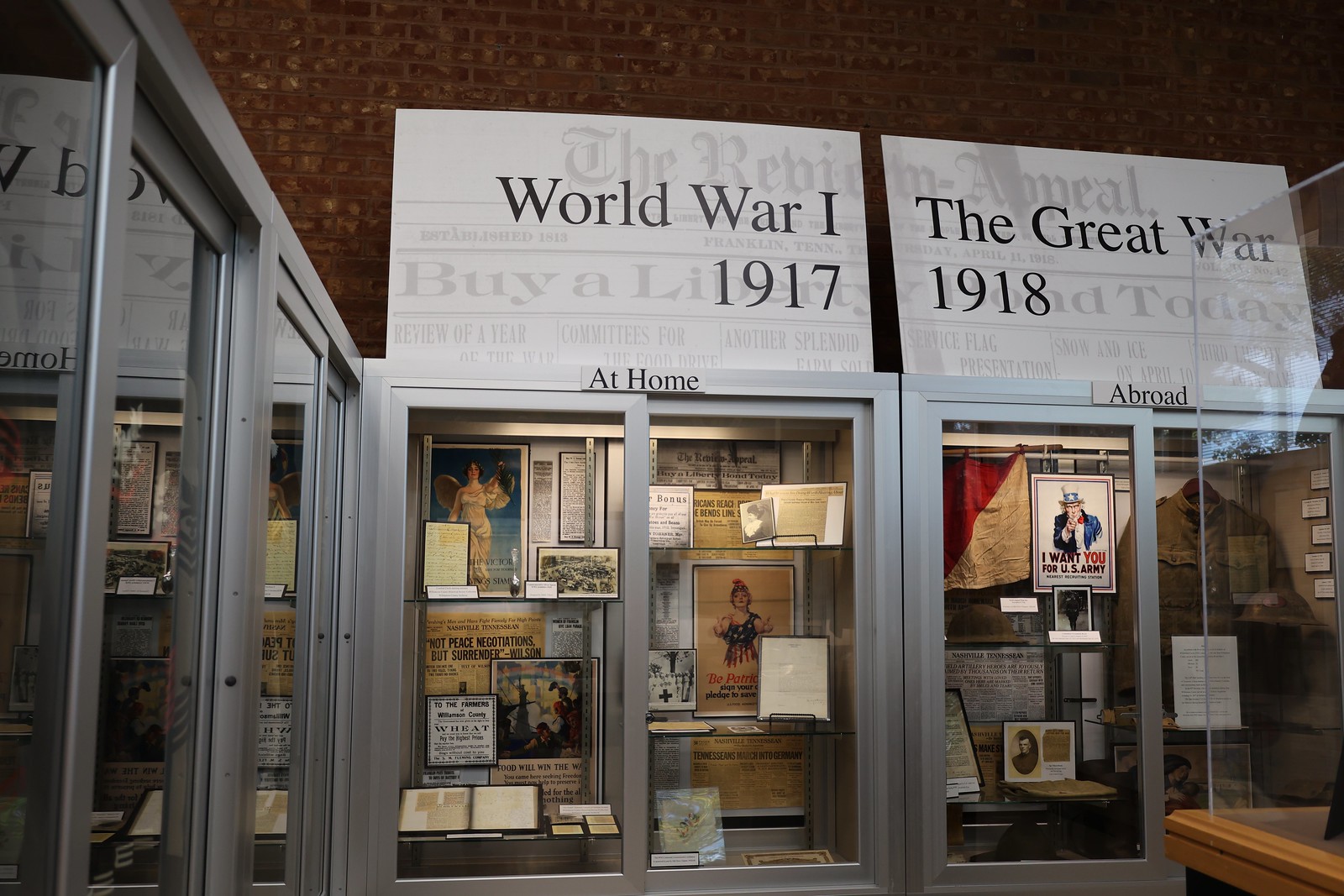This photograph depicts a museum exhibit focused on World War I, specifically highlighting the years 1917 and 1918. The exhibit is divided into two sections, with the left showcasing "At Home" and the right labeled "Abroad." Above the section on the left, a large white sign reads "World War I 1917," and it features artifacts such as newspaper clippings, political cartoons, posters, and documents, including one that dramatically states "Not Peace Negotiations but Surrender." The display also contains images, memorabilia, and more historical documents encased in glass. 

On the right, another large white sign announces "The Great War 1918," with a label on the exhibit case indicating "Abroad." This section contains a United States military uniform, an "I Want You for U.S. Army" recruitment poster, more newspaper clippings, and what appears to be a flag. Both sections are set against a prominent red brick wall. The entire scene is enclosed within the glass cases common in museum settings, creating a stark, historical narrative of the domestic and international fronts during World War I.